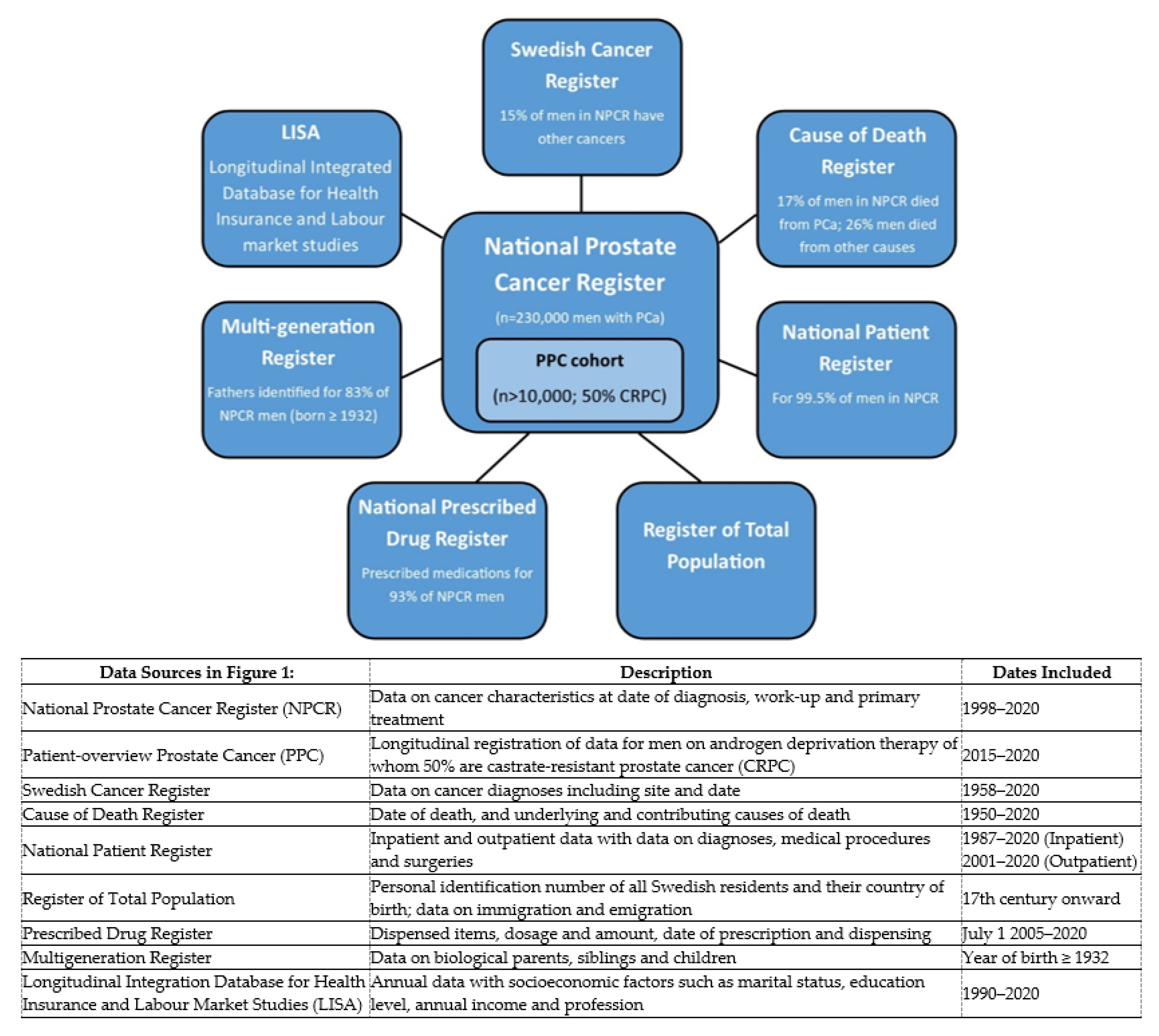The image depicts a comprehensive graphic showcasing data on the National Prostate Cancer Register (NPCR), containing a detailed bubble chart and a data table below it. The top section features a central blue rectangle labeled "National Prostate Cancer Register (N=230,000 men with PCA)," surrounded by six interconnected blue bubbles with white text and black outlines. Each bubble represents a different data source, such as the Swedish Cancer Register, Cause of Death Register, National Patient Register, National Prescribed Drug Register, Multigeneration Register, and LISA (Longitudinal Integrated Database for Health Insurance and Labor Market Studies), each providing relevant statistics and insights about the NPCR. A smaller light blue rectangle below the central bubble reads "PPC cohort, N > 10,000; 50% CRPC."

Beneath this visual, a nine-row black and white data table elaborates on the details of these data sources. The table's columns are labeled "Data Sources in Figure 1," "Description," and "Dates Included," offering in-depth descriptions and the timeframes of data collection. This image likely serves as an informative page from a textbook or medical journal, detailing the various components and associated statistics of the NPCR.